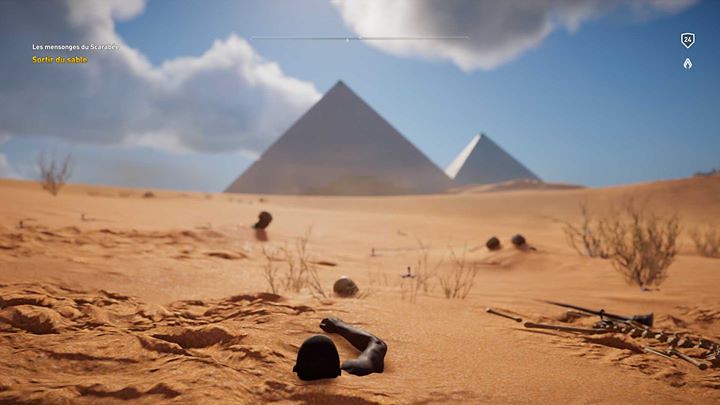This detailed digital screenshot from a video game captures a haunting desert scene under a medium blue sky adorned with large white and gray puffy clouds. In the background, two light gray pyramids rise against the horizon, with the larger one positioned centrally and a smaller one slightly to the right. The expansive foreground is dominated by a wide stretch of flat, light brown sand dotted with sparse, leafless bushes. Disturbingly, various human remains are partially buried in the sand: a skull whitening under the sun, four scattered skulls in the middle, and in the bottom right corner, a complete skeleton lies. Central to the scene is a man of apparent African descent, with his head and right arm emerging from the sand in a desperate crawl. Adjacent to this haunting tableau, there are guns with an ammunition belt. In the top corners of the image, French text reads "LES MONSONGES DU SCARAS" and possibly "ER," while the top right corner displays a diamond-shaped logo with the number 24 and another small white icon resembling a flame.